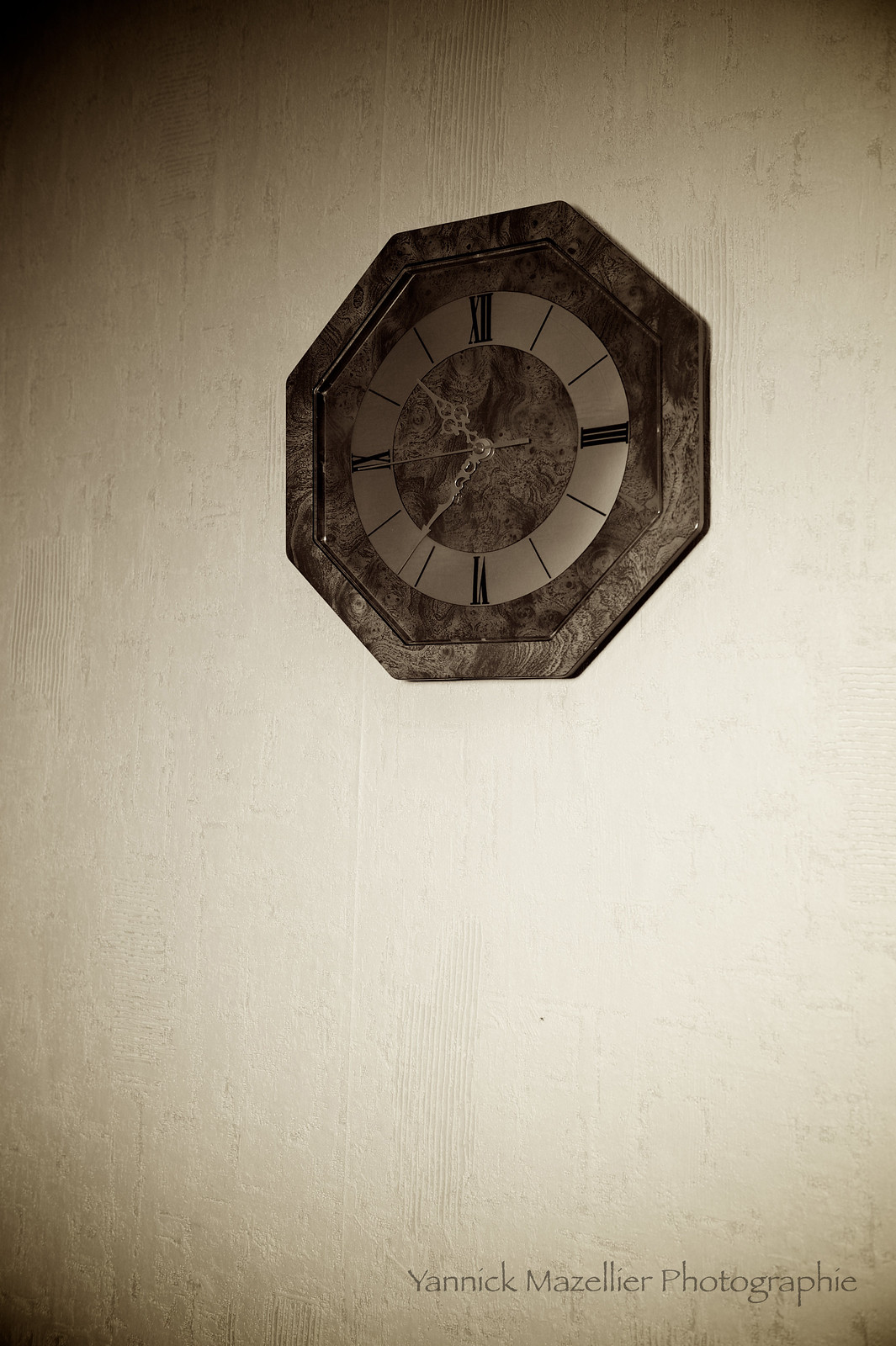Hanging prominently on a white painted wall, the hexagon-shaped clock immediately captures attention with its elegant and fancy design. The clock's face features striking black numerals that contrast sharply against the intricate hexagonal frame. Silver hands gracefully point to the time, standing out against the numerical background. The backdrop is a dark brownish hue with subtle lighter spots, enhancing the clock's sophisticated appearance. Notably, the clock occupies a significant portion of the wall, adding a touch of grandeur to the space. Beneath the clock, the text "Yannick Maziller Photography" is visible, crediting the talented photographer who captured this stunning image.